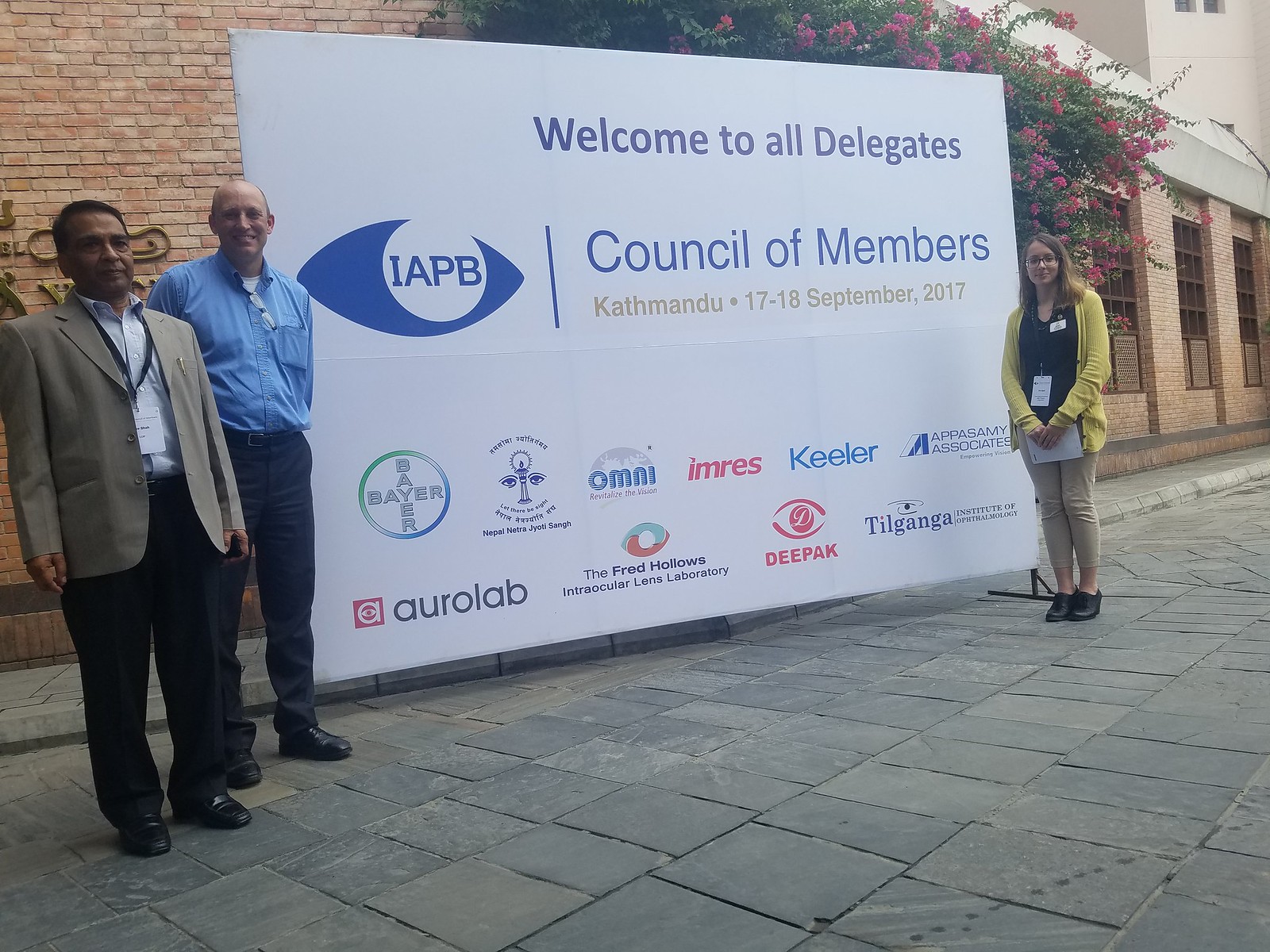The photo, taken outside along a sidewalk in front of a tan brick building, captures a scene featuring a large white cardboard sign adorned with blue text. The sign reads: "Welcome to All Delegates, IAPB, Council of Members, Kathmandu, 17-18 September 2017," and showcases a prominent logo of an eye with the letters "IAPB" typed into the iris. Below the main text, a series of logos representing various organizations, such as Healer, Deepak, the Fred Hollows Intracular Lens Laboratory, and Tilganga, are displayed. Behind the sign, a lush green tree with pink blossoms adds a touch of natural beauty to the setting.

Flanked by the sign, there are three individuals: two men on the left and one woman on the right. The first man, closest to the sign, is dressed in a blue long-sleeve shirt paired with dark pants and dark shoes. The second man stands beside him in a brown jacket over a light blue undershirt, also wearing dark pants and shoes. To the right of the sign, a woman is seen in a yellow jacket over a dark shirt, with light tan pants and dark shoes. These three people are framed between the vibrant sign and the blossoming tree, creating a balanced and engaging composition against the backdrop of the building.